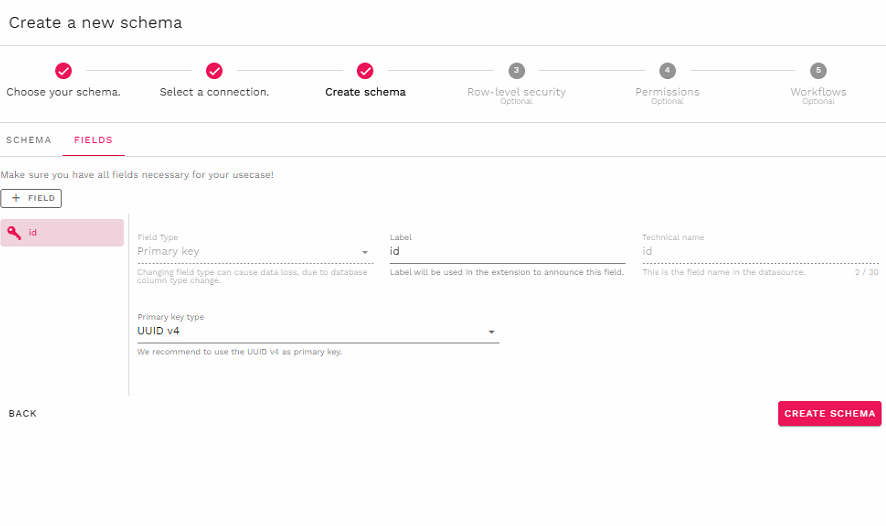The image is a screenshot of a website interface, predominantly featuring a clean, white background with pink and black accents for emphasis. At the top of the page, the title "Create a New Schema" is prominently displayed. Below the title, a series of steps are visually represented, each marked by a circle above it. Some of these steps have pink circles with white check marks, indicating completion. The completed steps are "Choose Your Schema," "Select a Connection," and "Create Schema."

The subsequent steps, which are not completed and are displayed with gray circles, include "Row Level Security," "Permissions," and "Workflows." Moving further down, you encounter the section titled "Schema and Fields," with a pink underline highlighting the "Fields" sub-section. Here, a note advises, "Make sure you have all fields necessary for your use case."

A box labeled "Field" follows, consisting of a pink box that denotes "ID" with a key icon beside it. This field is further detailed with several attributes:
- **Field Type**: "Primary Key"
- **Label**: "ID"
- **Technical Name**: "ID, UUID4"

Each attribute is accompanied by explanatory text:
- Under **Primary Key**, it warns: "Changing field type can cause data loss due to database column type change."
- For **ID**, it notes: "Label will be used in the extension to announce the field."
- Under **Technical Name**, it specifies: "This is the field name in the data source."
- For **Primary Key Type**, it recommends: "We recommend using the UUID as the primary key."

At the bottom of the section, there is a prominent pink button labeled "Create Schema."

This detailed layout provides a clear and instructional guide for users to create and define a new schema within the website interface.